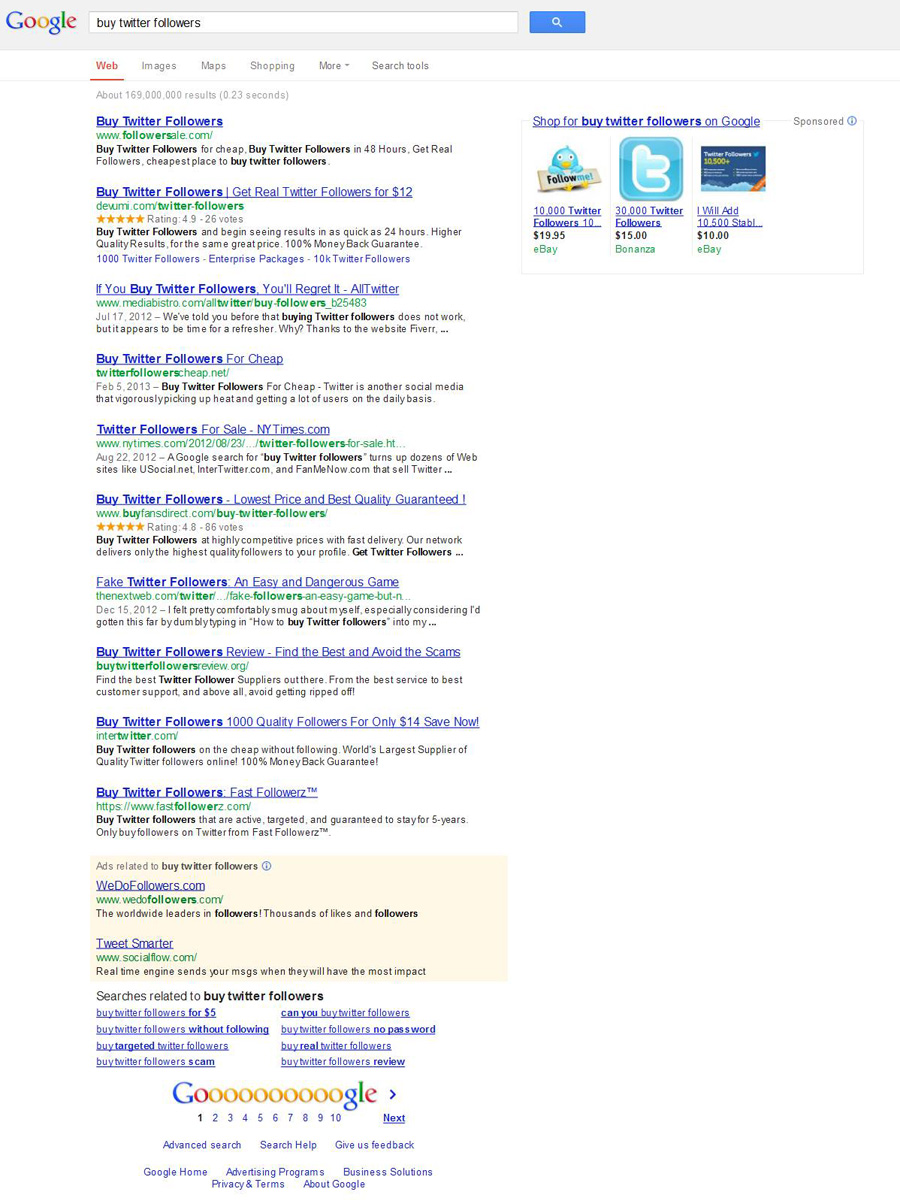A detailed screenshot of Google search results is displayed. At the top, there is a gray navigation bar. On the left side of the bar, the iconic Google logo appears, featuring the brand name in its signature multicolored letters. Adjacent to the logo is a white search field with the black text "buy Twitter followers" typed inside it. To the right of the search field, there is a small blue square containing a white magnifying glass icon, indicating the search button.

Beneath the navigation bar, a horizontal white menu bar shows various search categories labeled as "Web," "Images," "Maps," "Shopping," and "More search tools." The category "Web" is highlighted, indicating it has been selected. 

Below the menu bar, a status line indicates that there are approximately 100,609,000 results returned in 0.23 seconds.

The search results are listed in descending order, with the first result prominently displayed in blue font, reading "Buy Twitter Followers." Below this, a brief summary states: "Buy Twitter followers - Get real Twitter followers for $12."

The second result warns: "If you buy Twitter followers, you'll regret it."

Following this, the third result offers: "Buy Twitter followers for cheap."

The fourth result is identified as coming from the New York Times website, titled "Twitter followers for sale – NewYorkTimes.com."

The final listed result promises: "Buy Twitter followers - Lowest price and best quality, guaranteed."

All search results emphasize the various options and implications of purchasing Twitter followers.